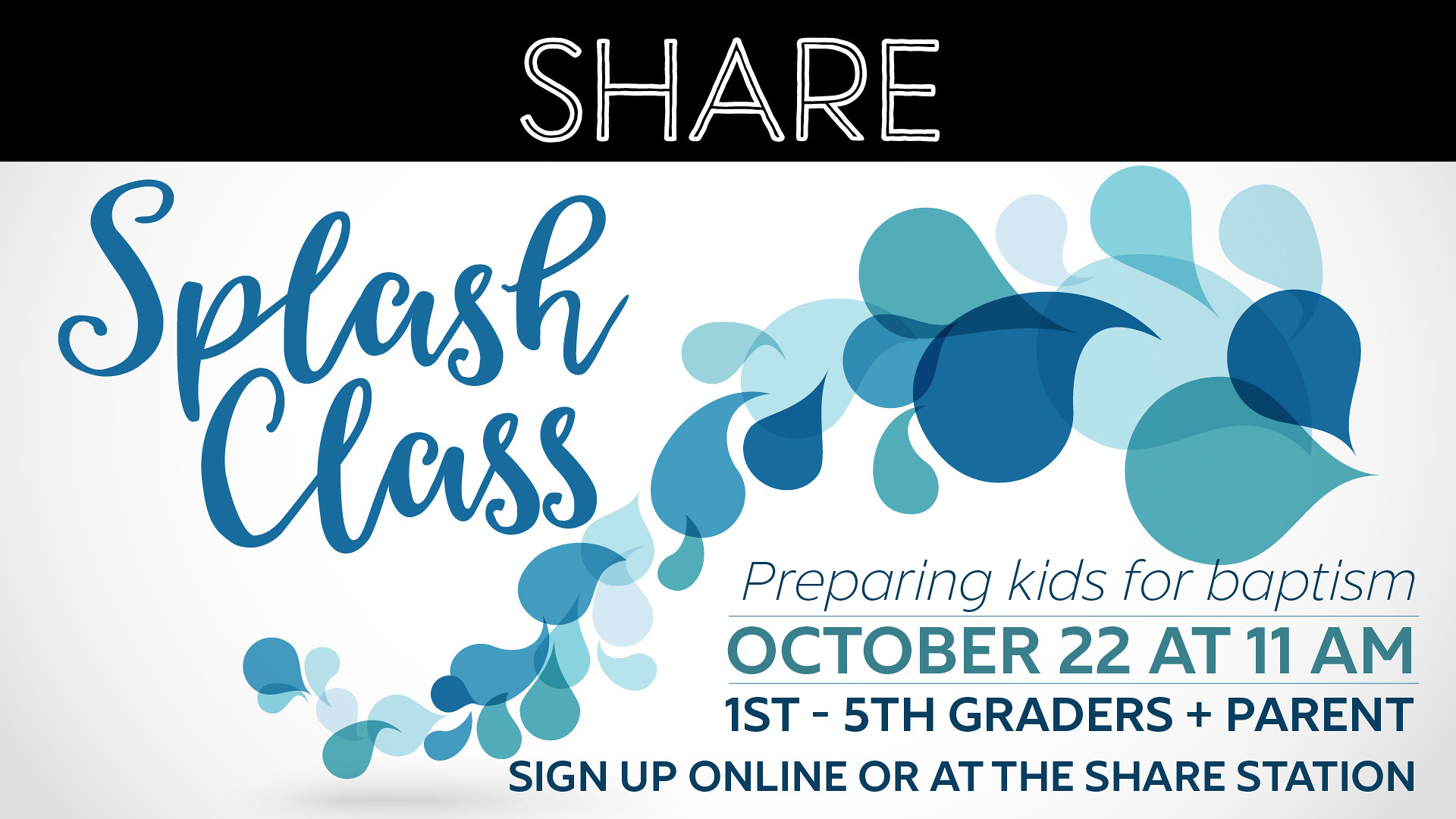This image is a vivid and elegant advertisement for an event from SHARE, featuring a harmonious blend of graphic design and typography. The top of the image sports a bold, horizontal black bar with the word "SHARE" prominently displayed in white shadowed letters. Below this, the background transitions to an off-white hue, adorned with various detailed shades of blue, featuring stylized cascading teardrop shapes.

In the upper left corner, the phrase "Splash Class" is illustrated in a bold, teal handwritten font, accompanying the teardrop designs that stretch from the right side of the image to the left in an S-shaped pattern. These design elements range in color from dark blue to aqua, enhancing the visual appeal.

Prominently positioned in the bottom right corner, the text reads: "PREPARING KIDS FOR BAPTISM" followed by "OCTOBER 22 at 11 a.m." in a seafoam green color. Below this, additional details include "FIRST TO FIFTH GRADERS PLUS PARENT" and "SIGN UP ONLINE or at the SHARE station," rendered in either very dark blue or black.

The image utilizes a cohesive color palette of black, white, turquoise, blue, light blue, and seafoam green, ensuring a visually striking and informative advertisement.